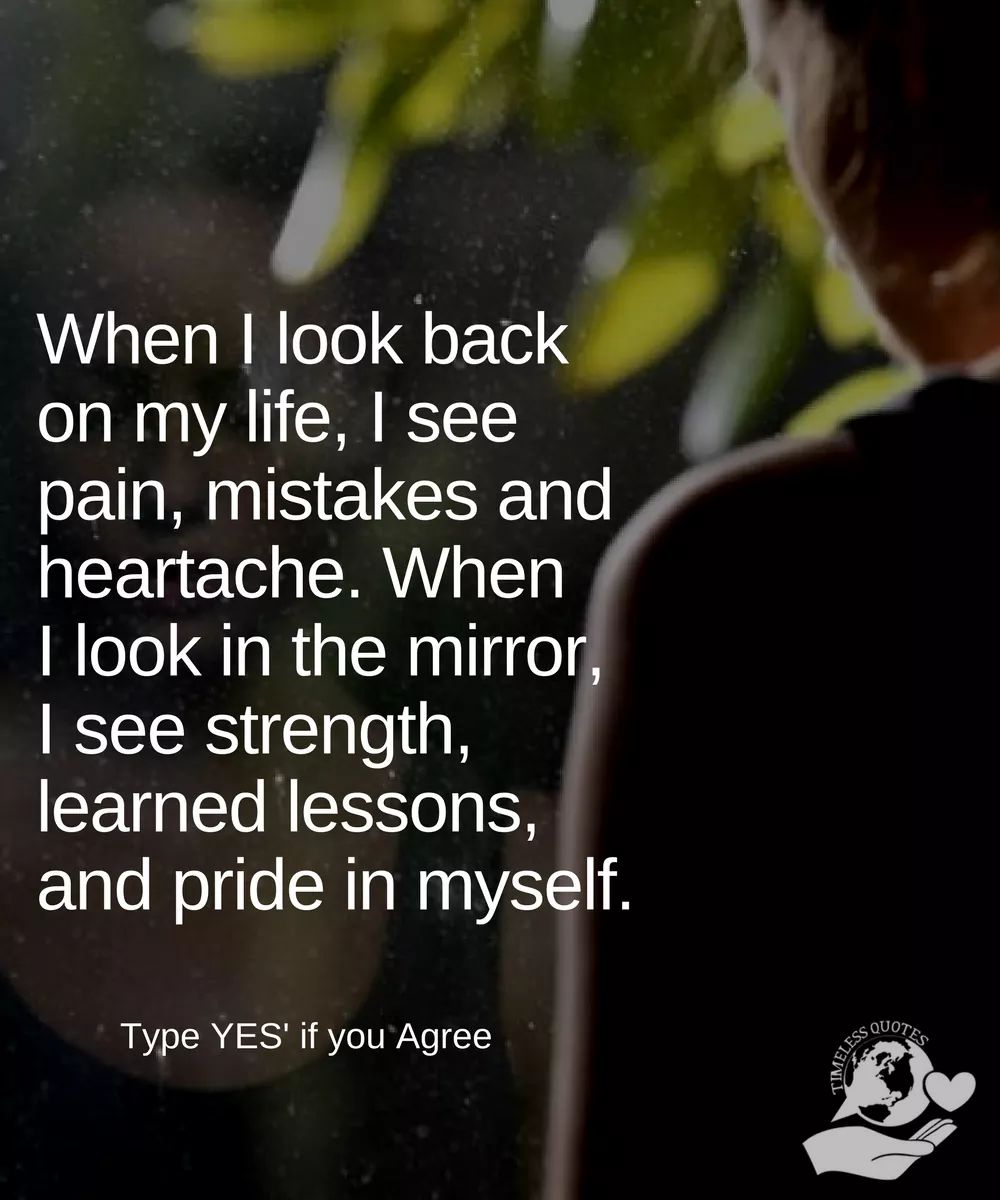The image resembles a stock photo typically used for motivational content on social media. It features a dark-toned background with a blurred, zoomed-in view of a person, likely a man or a woman, seen from behind. The person is positioned to the right and is partially cut off, showing only the back of their left shoulder, ear, and part of the head. A touch of green foliage is visible in front of them.

Dominating the image is a motivational quote in large white text that reads: "When I look back on my life, I see pain, mistakes, and heartache. When I look in the mirror, I see strength, learned lessons, and pride in myself." Below this, in smaller white text, it prompts viewers to "type YES if you agree."

The overall color palette includes shades of black, white, gray, tan, green, and yellow. In the bottom right corner, there is a logo featuring the words "timeless quotes" next to a globe and a hand holding a heart, reinforcing the motivational nature of the image.